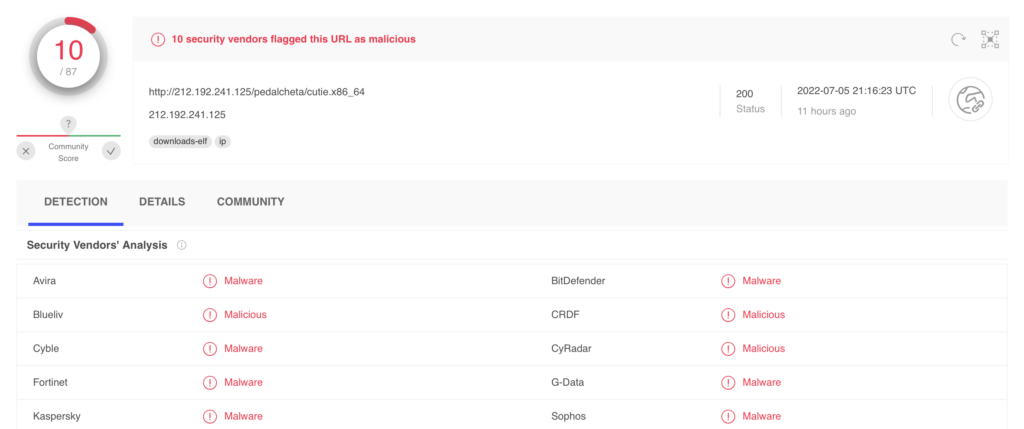**Detailed Caption:**

The image depicts a screenshot from a web security analysis platform. On the left side of the image, there's a circular graphic predominantly in shades of gray and white, featuring the number "10" written in red. A red bar partially overlays this circle. Adjacent to this, on the right side, there's a red circle containing an exclamation mark. The text next to it reads "10 security vendors flagged this URL as malicious."

Displayed below this warning is a URL, specifically an IP address, followed by the label "downloads.elf." The section titled "Detection details in community" is highlighted, with "Detection" underlined in blue, indicating it might be a clickable link. This section outlines multiple security vendors' analysis results.

The analysis lists several security vendors and their findings:
- **Avira**: Flagged as "malware," indicated by a red circle.
- **Blue IV**: Also listed as malicious.
- **Sybil**: Identified as malware.
- **Fort.net**: Detected as malware.
- **Kaspersky**: Listed as malware.
- **Bitdefender**: Also noted as malware.

All these detections are dated July 5th, 2022.